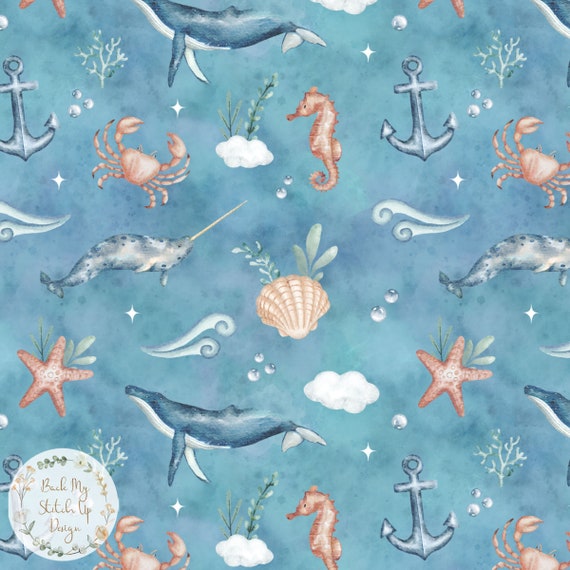This image showcases a whimsical nautical-themed fabric or material, possibly intended for bedding, curtains, or wallpaper. The design is vibrant and playful, dominated by a blue watery background adorned with light blue, silvery anchors, pinkish-beige crabs, and seahorses. Scattered throughout are various ocean elements including blue and white whales, pink and white starfish, beige seashells, and pieces of blue coral, giving the impression of an under-the-sea adventure. There's also green seaweed and bubbles rising from the ocean floor.

At the bottom of the image, there is a white circular label trimmed with greenery or garlands. Though the text within the circle is hard to decipher, it appears to read, "back my stitch up design," written in tan. This delicate label adds a touch of elegance to the playful and colorful marine tableau, which seems digitally crafted, enhancing its charming and imaginative appeal.